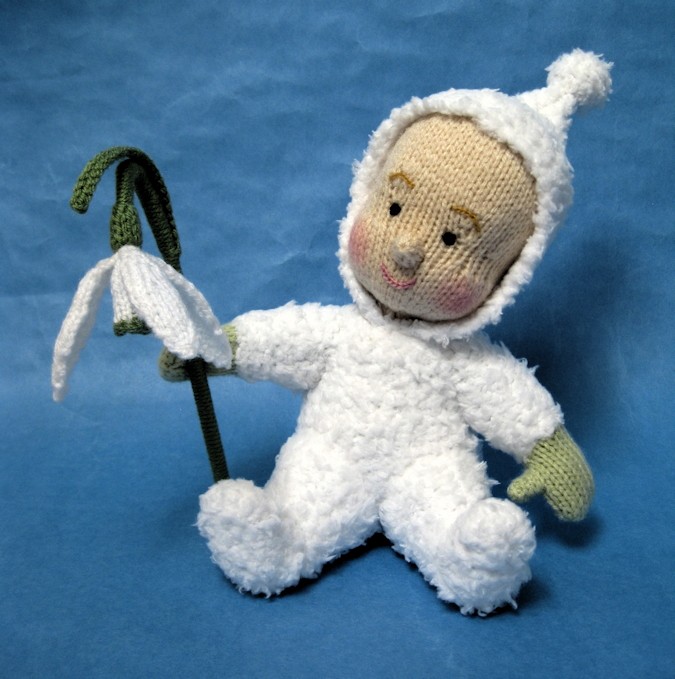This image showcases a handcrafted, crocheted doll meticulously placed against a slightly wrinkled, solid blue background. The doll, resembling a baby, is adorned in a white, fuzzy one-piece suit with a matching white hat that features a little tassel on top. The face of the doll is brownish-yellow with a warm, inviting expression characterized by pink blush on its cheeks, pink lips, brown eyebrows, and black eyes. The baby doll's head tilts slightly to the right while its gaze is directed to the left. It holds a delicate flower in its green-gloved right hand, the flower comprising a green stem and white petals that cascade down. This carefully arranged image not only highlights the skillful craftsmanship of the crocheted item but also evokes a heartwarming, winter-ready aesthetic through the doll's attire and accessories.